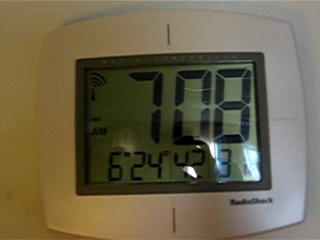This photograph showcases a white-bodied electronic device with a central black digital display, bordered by a gray square frame. At the bottom of the device, "Radio Shack" is printed in gray font. The black digital screen prominently displays the text "AM" in black font, along with the time "7:08." Additional numbers visible on the display include "6," "24," "42," and "3," though there is some light glare causing slight distortion at the bottom of the screen. The device's reflective surface adds to the image complexity. The white body of the electronic device is positioned against a matching white background, making the overall image sleek and cohesive, notwithstanding the minor glare issue.